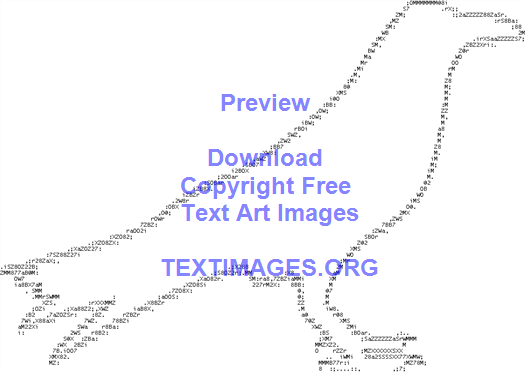The image is a bird, specifically a side profile outline of a crow-like bird facing towards the right. The entire silhouette of the bird is formed by various computer-generated text, primarily in black. The background of the image is completely white, creating a stark contrast. Prominent blue text is superimposed over the bird, reading "Preview," "Download," "Copyright Free," "Text Art Images," and "textimages.org," positioned centrally from the top to just above the bird’s legs. The bird’s outline reveals a narrow body, thick legs with toes pointing towards the bottom right corner, a long beak at the top right, and delineated tail feathers extending towards the bottom left corner. The bird’s wings appear folded and are not distinctly visible, contributing to the minimalist, text-based sketch.